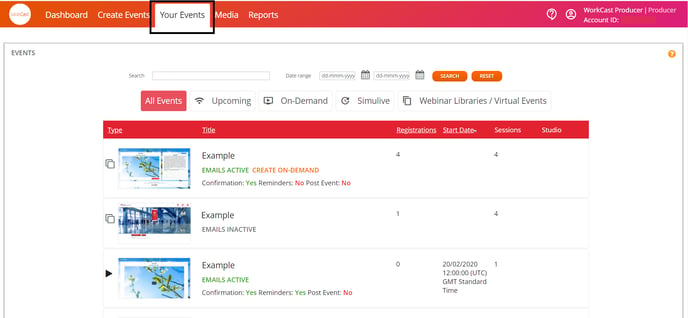The image depicts a comprehensive dashboard interface. On the left side, there is a white circular icon with an undecipherable orange inscription and an orange strip along the top. To the right of this icon, there are several menu options listed vertically: "Dashboard," "Create Event," "Your Event," "Media," and "Reports." 

On the right side of the dashboard, the menu options include "Work Cart," "Producer," "Producer," "Account," and "Settings." Notably, the "Your Event" option is highlighted with a white background, black font, and a black rectangle outline, while the other options feature an orange background with white font.

The top-left corner of the page indicates that the user is currently on the "Events" page. Directly below this, there is a search bar without any input data. Adjacent to the search bar, there is a "Date Range" field followed by two data fields each accompanied by a calendar icon. Further to the right are two buttons: an orange "Search" button with white text and an orange "Reset" button also with white text.

Below these search functionalities, a series of tabs or buttons is listed horizontally. They include "All Events," "Upcoming," "On Demand," "Simulive," "Webinars," "Libraries," and "Virtual Events."